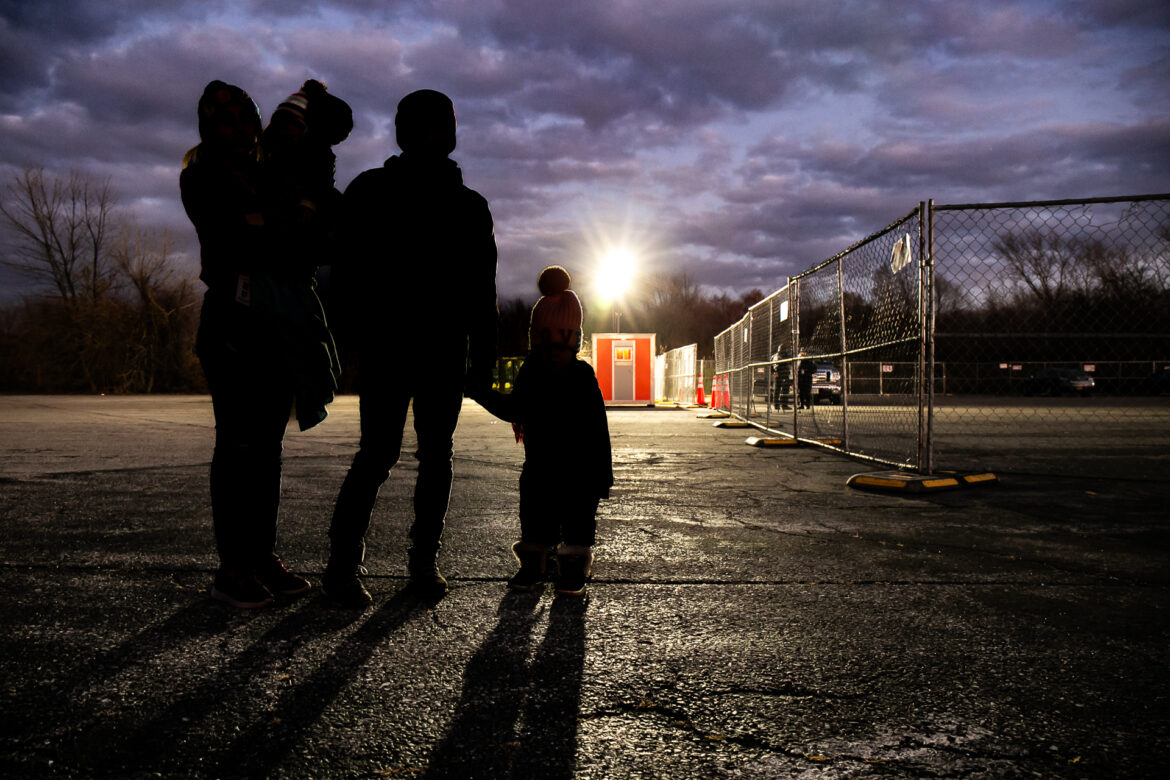The image is a horizontal rectangular photograph captured at dusk, depicting a family of silhouettes standing on a worn, cracked asphalt lot as the sun sets behind a small red shed with a gray door. The family consists of two adults and two children; one adult holds a child in their arms while the other holds the hand of another child. The ground is illuminated by a bright spotlight from a tall rod attached to the shed, casting the family in shadow. A chain-link fence stretches from where the family stands to the shed, and in the background, two men in dark uniforms stand next to a dark SUV near a gap in the fence marked by three orange traffic cones with silver reflective stripes. The sky above is mostly cloudy with a hint of blue, and a large patch of yellow from the setting sun.